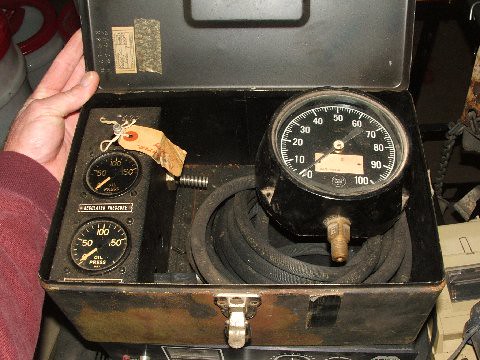The image shows the interior of a metal box with its top lid open. Inside the box, on the right side, there is a circular gauge with a black face and white numbers ranging from 0 to 100. The needle of the gauge is pointing at 0, and there is a white circle in the center of the needle. Beneath the gauge, there is a white-colored rectangle. Below the gauge, a dusty, copper-colored inlet port is visible, surrounded by a black hose featuring several circular patterns.

On the left side of the box, there are two more dials. The upper dial has a black center and displays faded numbers that appear to range from 50 to 100. The yellow-colored needle of this dial points downwards to the left. The lower dial resembles the upper one but has brighter, more legible numbers. 

Outside the box, on the far left, an arm clothed in a red long sleeve extends towards the box. The hand is visible, with the thumb holding open the lid and the index and little fingers partially obscured behind the box.